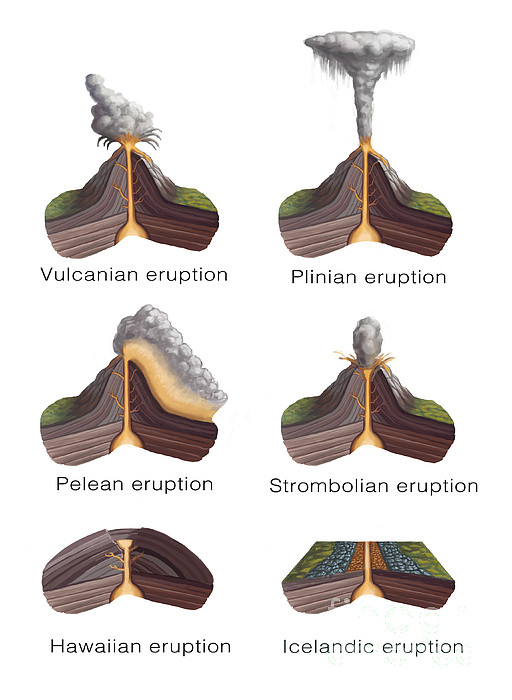The image features a series of six detailed drawings depicting various styles of volcanic eruptions, all set against a white background. Arranged in two columns and three rows, each drawing provides a cross-sectional view of a volcano, showcasing the point of eruption and the resulting plume, if any. The top row includes, from left to right: a Vulcanian eruption, illustrating lava and smoke emerging explosively from inside the mountain; a Plinian eruption, characterized by an enormous mushroom-shaped cloud of ash and smoke reaching high into the air; and a Pelee eruption, where lava flows down the mountain sides amidst accompanying smoke. The second row showcases, from left to right: a Strombolian eruption, marked by a q-tip shaped burst of smoke; a Hawaiian eruption, presenting only the flow of lava without any smoke; and finally an Icelandic eruption, similar to the Hawaiian type, showing lava flow with no accompanying smoke.